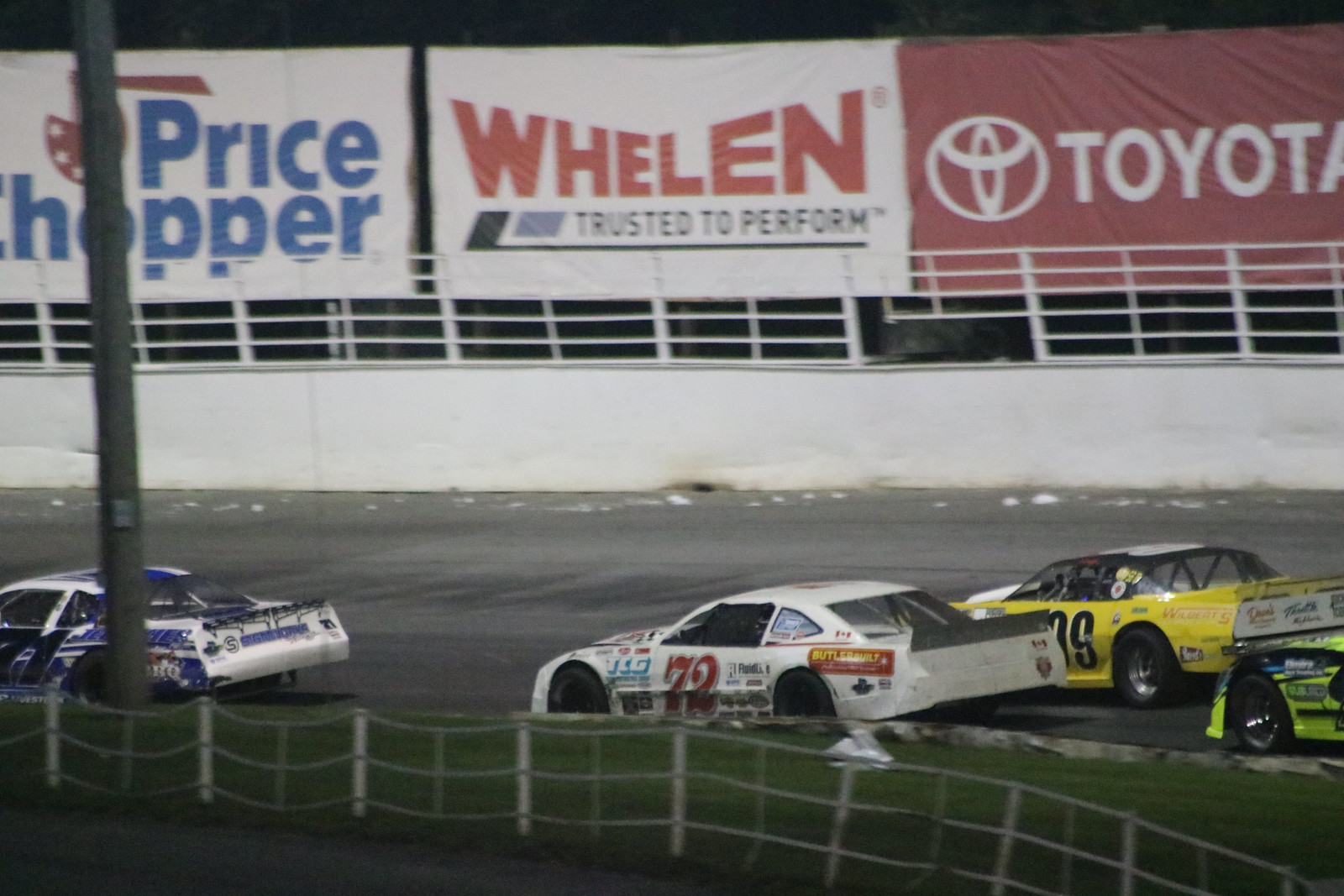The image captures an outdoor car race on a racetrack, featuring four cars navigating a bend. In the lead is a white car with extensive blue trim marked with the number 71. Trailing it is a white car with the red number 72. To the right of this car is a yellow vehicle with black lettering, although its number is obscured. The front portion of a neon yellow car is also visible. The racetrack itself is a mix of gray and black, bordered by a white rail fence. Beyond the track and fence, there is another steel fence, with three large advertising banners mounted on it. The left banner displays "Price Chopper" in blue letters, the middle one reads "Wheelan" in red letters, and the right one shows "Toyota" in white letters along with its logo. A patch of green grass with a telephone pole is visible in the foreground to the left. The overall scene is somewhat blurry and dark, creating a slightly grayish hue over the photograph.